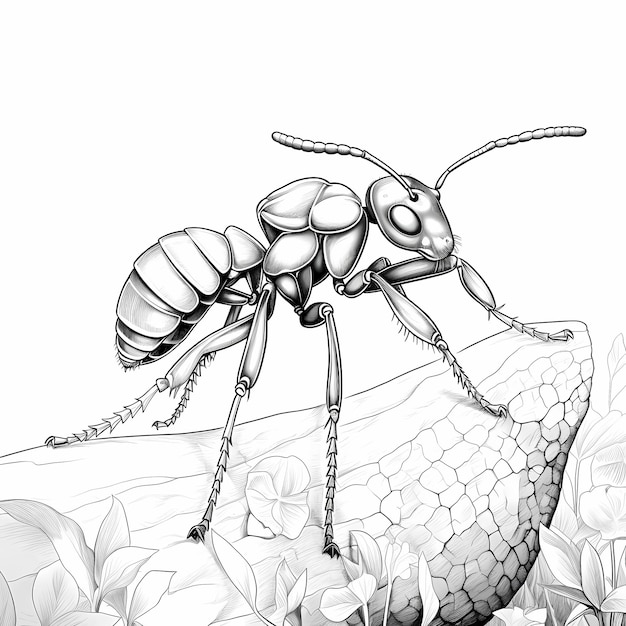This highly detailed black-and-white digital rendering captures a close-up, almost face-to-face perspective of an intricately detailed ant. The image showcases the ant standing on a textured piece of tree bark, possibly rock or wood, which is adorned with numerous cracks and fissures, adding to the realism. The ant’s body is rendered with precision, highlighting its segmented form, including its head, thorax, and abdomen. You can clearly see its distinctive features such as its two segmented antennas, beady eyes, and mouthparts lined with tiny hairs. The legs, covered in fine prickling hairs, emphasize the alien-like appearance of the creature. The ant is oriented from right to left, revealing only its right eye in this stance. Surrounding the ant, at the base, are black-and-white flowers and plant leaves that may resemble petunias or pansies, which add a naturalistic foreground to the composition. The background above is left white, enhancing the focus on the detailed foreground.